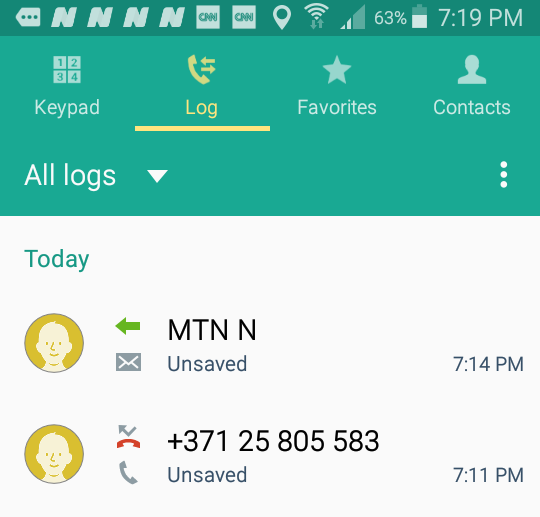**Detailed Caption:**

This image is a detailed screenshot, specifically a cropped section displaying a mobile phone's call log interface. 

At the top of the screenshot, a dark sea-green bar stretches across the background, indicating an active status bar loaded with various notifications. Starting from the left, there are three vertical dots, followed by a distinct 'N' symbol which repeats three more times. Next, there's a CNN logo inside a square icon, followed by another identical CNN logo. To the right of these, the location symbol is visible, indicating that location services are active. Beside that, the Wi-Fi symbol shows full connectivity, while the cell phone signal strength is displayed as two out of four bars. Adjacent to this information, the battery percentage is at 63%, next to a horizontal-vertical battery icon. On the far right, the time is displayed as 7:19 PM.

Beneath this status bar, we move into the call log's navigation header, which features a lighter variant of the sea-green background. This section's text color is a very light hue, almost white with a subtle tint of the sea-green color. From the left, the navigation options include 'Keypad' with a keypad icon, 'Log' marked with a yellow-highlighted phone icon with arrows, signifying the active section. Next, 'Favorites' is denoted by a star icon, and 'Contacts' displays a person-shaped icon.

On the next row, the leftmost label reads 'All Logs' with a downward-facing arrow, and on the far right is a three-dot menu button. Following this header, the background transitions to a light gray shade, designated for the call log's main content area.

In the call log section, the label 'Today' in sea-green color marks the timestamp of the listed calls. The first entry features an avatar of a generic man, illustrated in a light yellow vector style against a dark yellow background with a black outline. To its right, a green arrow icon points left, followed by a message icon. The text to its right reads "MTN n" above the word "unsaved," and the time stamp "7:14 PM" is positioned on the far right.

The second call log entry replicates the same avatar. To its right, a red missed call icon appears, showing a phone with an arrow. Below this, a phone icon precedes the number +371 25 805 583, followed by the word "unsaved." The call time for this entry is stamped as "7:11 PM." The image ends here, encapsulating the described elements.